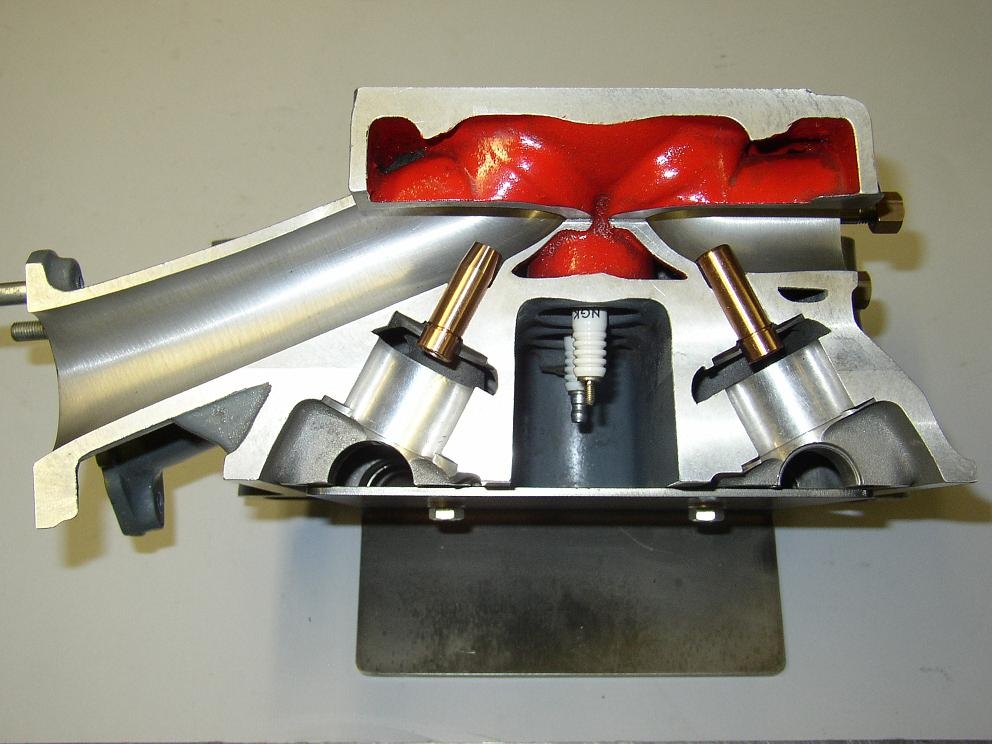This detailed image shows a meticulously crafted cross-section of a metallic twin-cylinder engine part, likely the upper portion of an engine. The majority of the machinery is composed of thick, silver-gray metal, highlighting its sturdy construction. Resting on a flat, rectangular metal plate, the engine part features two prominent piston-like cylinders positioned on either side. A clear focal point is the top section, which includes a vividly painted dark orangish-red chamber, possibly filled with latex or gel. 

Beneath this red chamber hang two visible white NGK spark plugs, indicative of the engine's ignition system. Along the left-hand side, there is a large exposed metal tube or intake pipe that extends upward into the chamber, suggesting a crucial role in air or fuel intake. The image reveals that the mechanical object appears to be cut in half, suggesting the visible internal components such as bolts, screws, and internal tubing. The object, likely photographed on a white or light gray surface, is a modern depiction of engine engineering, revealing intricate internal structures often concealed within a finished engine.